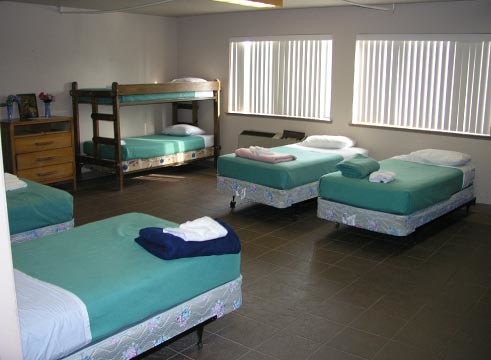The image depicts a room reminiscent of a hostel, sick ward, or barracks with six twin beds scattered throughout the space. The beds, including a wooden-framed bunk bed positioned in the corner, are uniformly dressed in teal-green bedsheets and feature white pillows. Some beds have neatly folded clothing on top, while others do not. Notably, there is a chest adorned with what appears to be a religious picture flanked by flowers near the bunk bed. The room is illuminated by natural light streaming through two large windows with shades on the back wall, adding to the sense of openness. The beds rest on a floor of brown tile, while the white walls create a stark, clean environment. Among the beds, four are aligned along the walls and two can be partially seen in the foreground. The overall setting suggests a communal living space designed for multiple occupants.